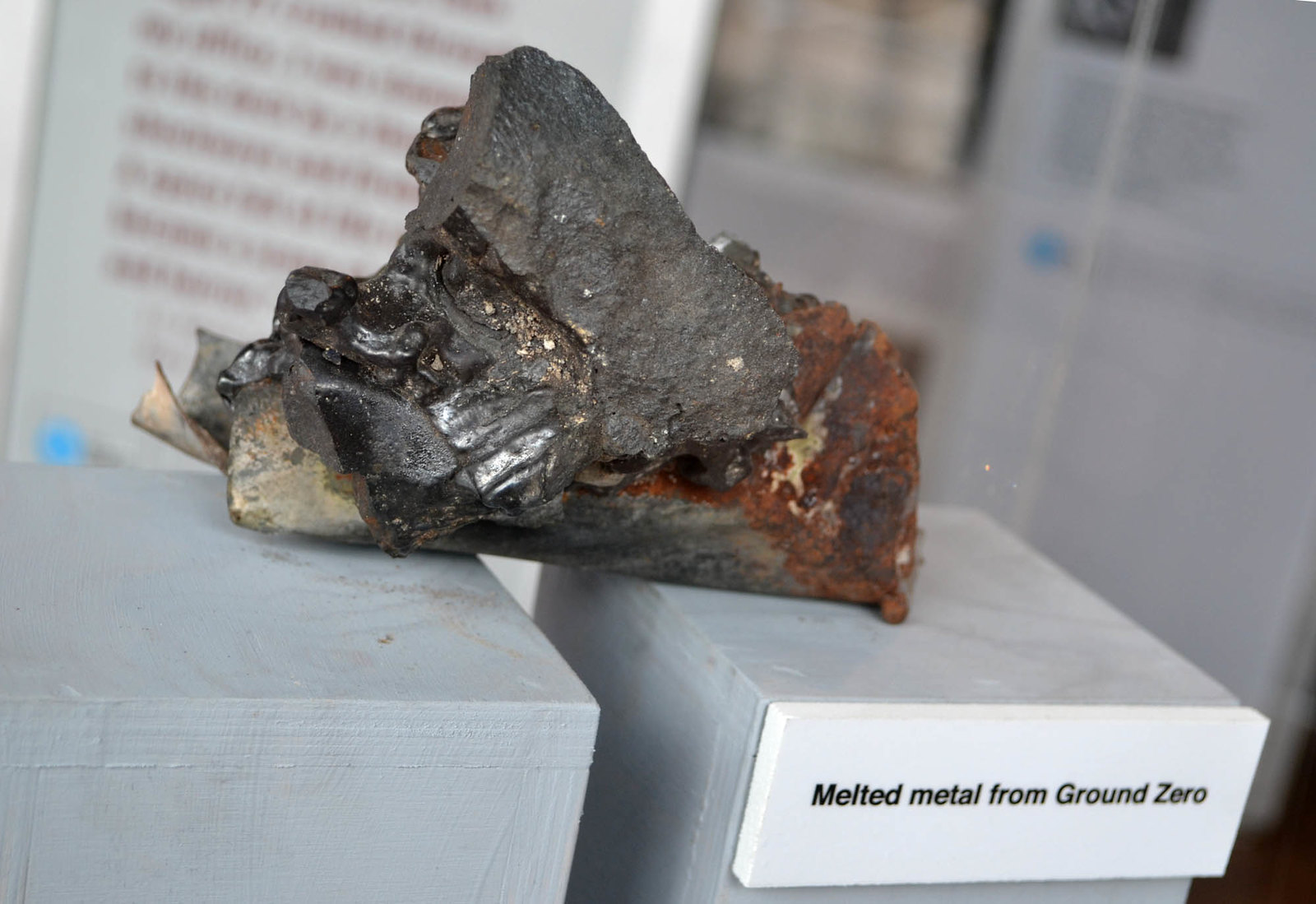The image depicts a close-up of a jagged, burnt, and twisted piece of metal, displayed prominently in a museum. The metal, likely from the September 11th, 2001 terrorist attacks at Ground Zero, rests on two small light blue pedestals made of cement or wood, which are split in the middle. Numerous colors and textures are apparent on the metal; it has dark gray sections, shiny black marble-like areas, and rusted parts with orange and yellow hues. A small white sign with black text beneath the metal reads, "Melted metal from Ground Zero." The background features walls with informational write-ups, indicating the educational context of the display. No glass cover is visible, but it might be due to the photo's angle. This poignant exhibit piece serves as a tribute to the tragic events and the lives lost on that day.